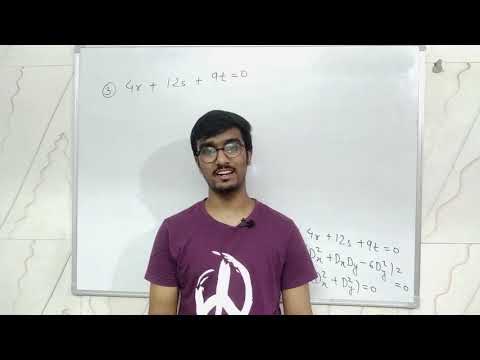This is an image, possibly a screenshot from an online video, of a young Indian man standing indoors in front of a whiteboard with a shiny silver frame. He has short black hair, round glasses, a thin black mustache, and a small goatee. He is wearing a short-sleeved purple or maroon t-shirt featuring a white peace sign in the middle and has a small black microphone clipped to the upper right corner of his collar. He is standing against a background of a white wall with gray squiggly lines, which also casts a shadow behind him. The whiteboard has mathematical equations written in black marker: one equation, "4R + 12S + 90 = 0", is prominent at the top left marked as "number three," while more equations are partially visible at the bottom right, obscured by the man. He is smiling at the camera, possibly mid-speech, suggesting he might be a teacher or lecturer in a casual setting. The image quality is slightly pixelated with a black border at the top and bottom, hinting that it might be a grab from a video with less than optimal resolution.